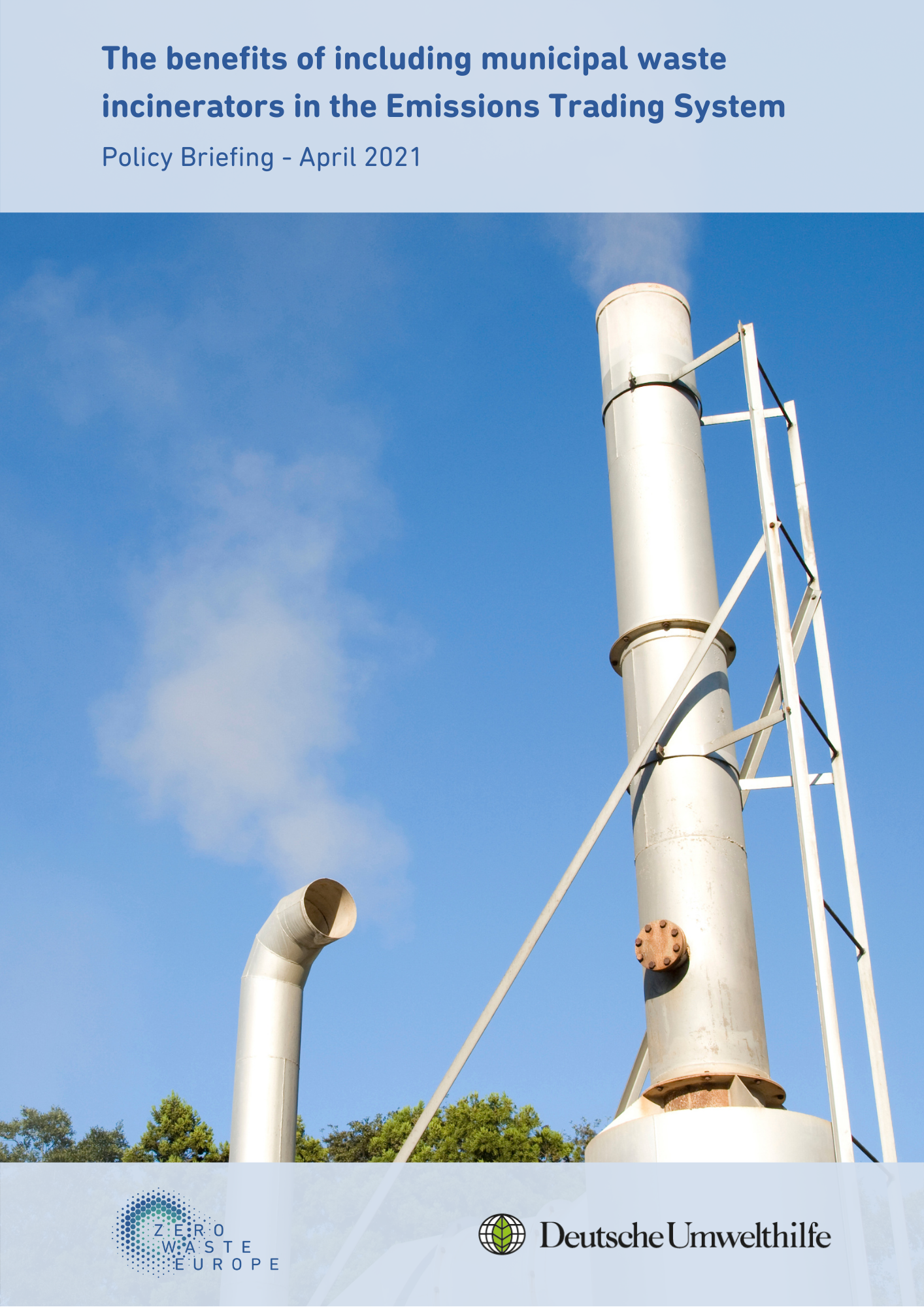The image features two prominent smokestacks, part of a municipal waste incinerator, set against a clear blue sky with a backdrop of green trees at the bottom. One smokestack, on the left side, is shorter and curved towards the right, while the taller smokestack on the right has a ladder running up its side and is surrounded by metal rods for stability. Both smokestacks are emitting light-colored smoke. At the top of the image, a rectangular section contains the title "The Benefits of Including Municipal Waste Incinerators in the Emissions Trading System" in blue sans-serif font, followed by "Policy Briefing - April 2021". At the bottom, in another light-colored rectangular section, logos for "Zero Waste Europe" on the left and "Deutsche Umwelthilfe" on the right are displayed.